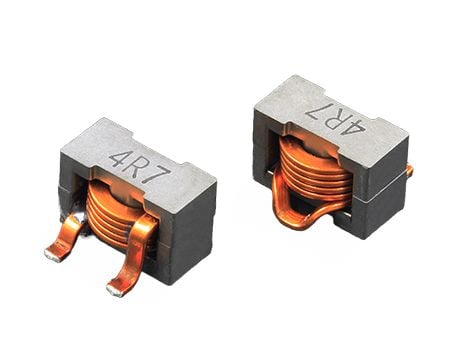The photograph displays two nearly identical metal rectangular objects against a completely white background. Each object has "4R7" engraved on the top and contains intricate gold or copper wiring inside. The objects are positioned at slightly different angles, giving the impression of one item viewed from two perspectives. The left object is a gray oblong square with two copper connectors protruding from the side, suggesting the beginning and end of the wrapped wire inside. In contrast, the right object shows a more circular arrangement of the wiring, tucked neatly with connected ends. Both items appear to be some type of electrical components, characterized by the metallic and copper elements visible through an opening on the top.